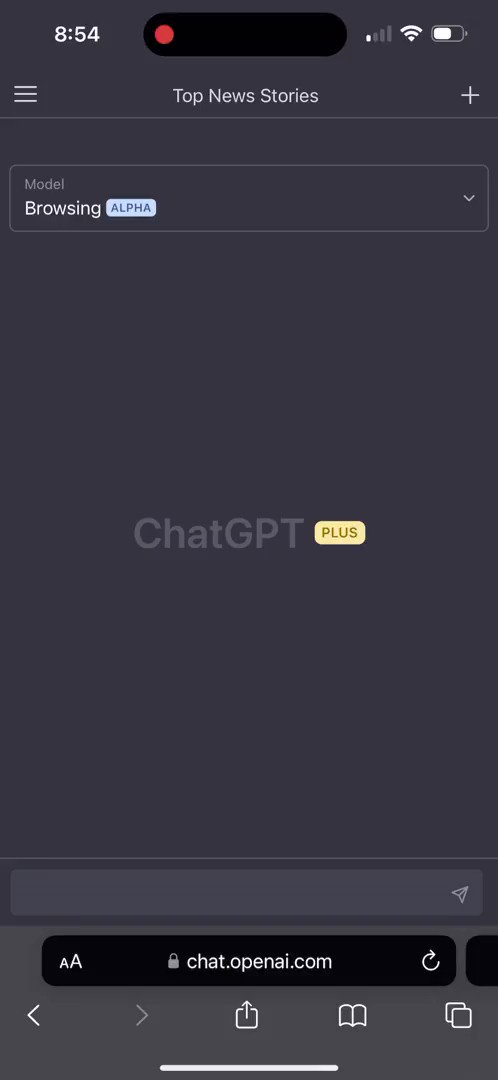Here is the cleaned-up and detailed caption for the described image:

---

The image depicts a cell phone screen displaying an interface related to browsing and communication. At the top left corner, the screen shows three bars indicating cell signal strength, next to a Wi-Fi symbol, and a battery icon that is approximately half full. 

Below these icons is a black search field with a distinctive red circle on its left side. The search field's background is predominantly dark slate gray, featuring the text 'Top News Stories' in white. Just above the search field are three horizontal lines, often used to represent a menu, and a plus sign on the right side.

Directly below the search field is a noticeable line separator, followed by a dropdown menu labeled 'Model Browsing Alpha,' suggesting an option for selecting different browsing models. 

Further down is an open field, primarily dedicated to 'Chat GPT Plus,' where 'Plus' is highlighted within a yellow rectangle with brown lettering. Another line separator follows beneath this section.

The next visible element is a rectangle icon that appears to resemble a paper airplane. Immediately below this icon is a thick black bar reading 'locked chat.openai.com.' The left side of this bar features a small 'A' and a large 'A,' symbolizing text size options, while the right side displays what seems to be a refresh symbol.

At the bottom of the image, on a dark gray background, there are navigation icons, including left and right arrows for going back and forward, a square with an upward-pointing arrow representing sharing options, and an open book icon, likely indicating a library or reading mode feature.

---